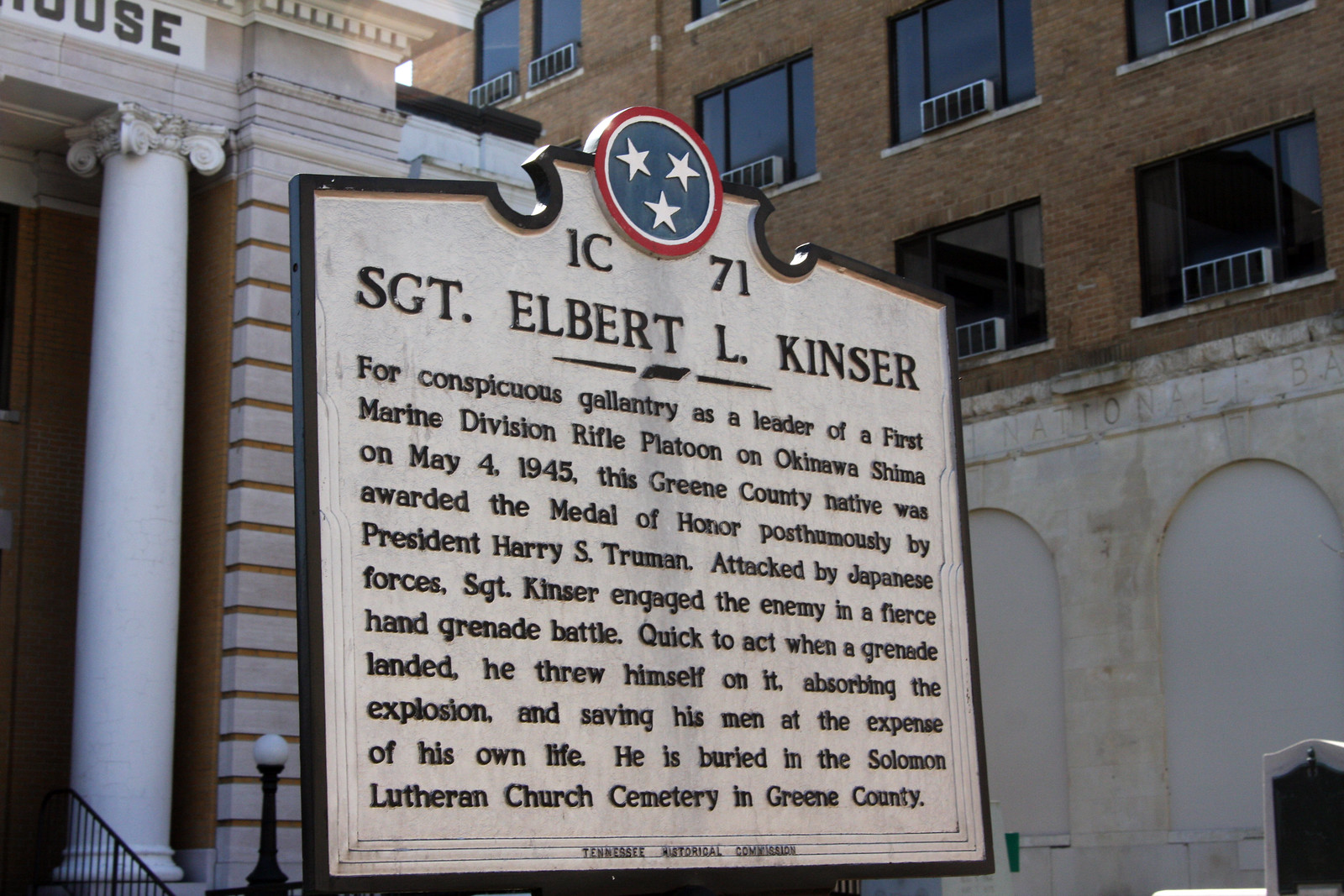The photograph, taken outdoors in a city setting, captures a close-up of a historical sign prominently positioned in the center, with tall buildings partially visible behind it. On the left, there is a building featuring a gigantic white pillar and partially visible text appearing to spell "house" at the top left-hand corner. The right side reveals a large brick building with multiple rows of windows. The sign itself displays a red-edged circular logo with a blue center that contains three white stars, surrounded by white and red rings. The text on the sign reads: "1C71 SGT Albert L. Kintzer. For conspicuous gallantry as a leader of the 1st Marine Division Rifle Platoon on Okinawa-Shima on May 4, 1945. This Greene County native was awarded the Medal of Honor posthumously by President Harry S. Truman. Attacked by Japanese forces, Sergeant Kintzer engaged the enemy in a fierce hand-grenade battle. Quick to act when a grenade landed, he threw himself on it, absorbing the explosion and saving his men at the expense of his own life. He is buried in the Solomon Lutheran Church Cemetery in Greene County."